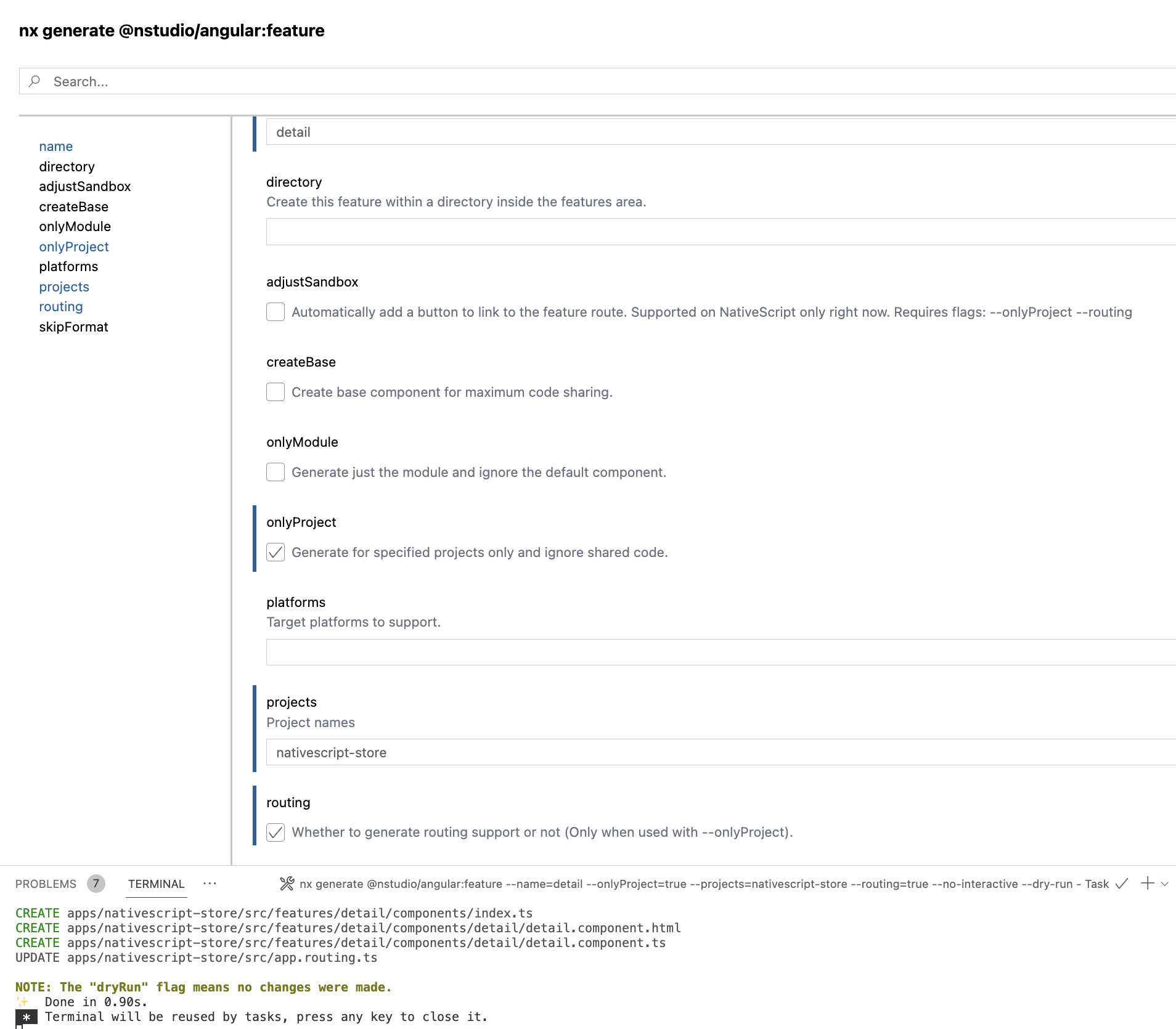This image is a screenshot of settings in a mobile app or website interface. The background is predominantly white, and the upper left corner features a text label in black font that reads “nx generate @nstudio/angular:feature.” Directly below this label is an elongated search field, centrally displaying the word “search” in grey font and accompanied by a small grey magnifying glass icon on the left side.

Positioned vertically on the left side is a detailed menu with multiple options including: 
- Name
- Directory
- Adjust Sandbox
- Create Base
- Only Module
- Only Project
- Platforms
- Projects
- Routing
- Skip Format

To the right of this vertical menu, detailed settings are displayed. At the top, there is a section labeled "Directory," which instructs users to create the feature within a directory inside the features area. This section features a text box for input. Below this is a section titled "Adjust Sandbox" with a description that mentions the automatic addition of a button to link to the feature route, specifying that it is supported only on NativeScript for now and requires flags such as “--onlyProject” and “--routing.”

Further down, there is another section labeled "Create Base," describing the creation of a base component for maximum code sharing. 

Overall, the screenshot captures a comprehensive view of the feature generation settings, providing users with various configuration options for their project.